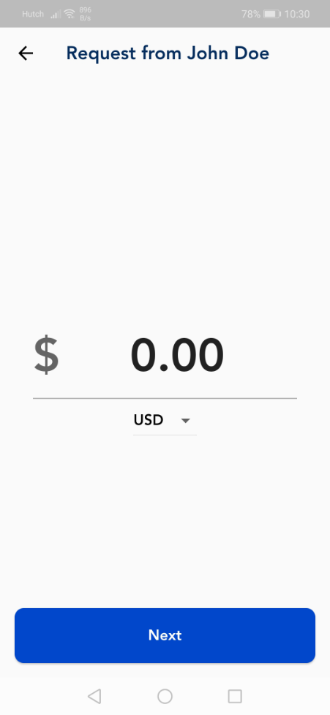The image displays a smartphone screen with a gray header area at the top which contains several icons, including an indistinct battery icon due to blurriness. Below this header, there's a prominent white section. On the left side of this section, a black arrow points to the left. Next to the arrow, dark blue text reads "Request from John Doe," positioned above a numerical value "$0.00." 

Beneath this, a light-colored horizontal line runs partially across the screen, stopping short of both the left and right edges. Below the line, the text "USD" appears, accompanied by a drop-down button. 

At the bottom of the screen, a large blue rectangular button bears the label "NEXT." Underneath this, there are three geometric icons: a triangle, a circle, and a square. The entire composition is set against a backdrop of significant empty space around the numerical values, emphasizing the central content.